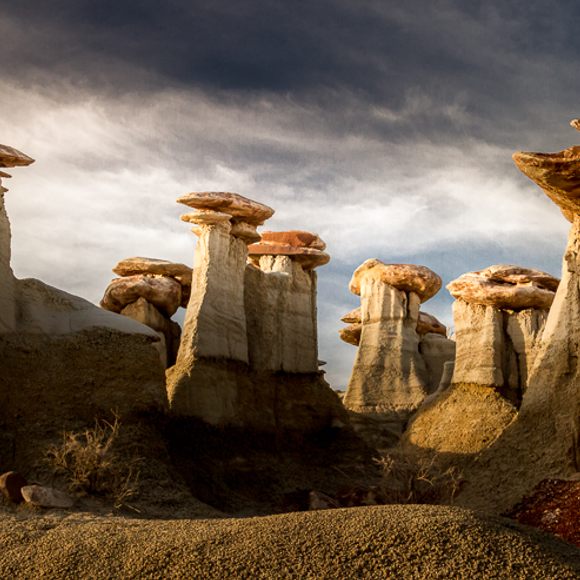This image showcases an array of tall, natural stone structures set against a gloomy, darkening sky filled with gray and blue clouds, evoking a brooding atmosphere. These towering stone formations resemble giant mushrooms with their thick, robust rock columns leading to broader, cylindrical tops. The varying colors along their heights suggest different historical sediment levels and watermarks. The ground below is a dark green, grassy expanse, contrasting with the brownish tones of the rock columns, which stand at an impressive height of around 15 to 20 feet. The stones are scattered and predominantly grouped in pairs, casting elongated shadows across the earth. This striking scene, reminiscent of Stonehenge, highlights the magnificent outdoor exhibits crafted by Mother Earth herself.